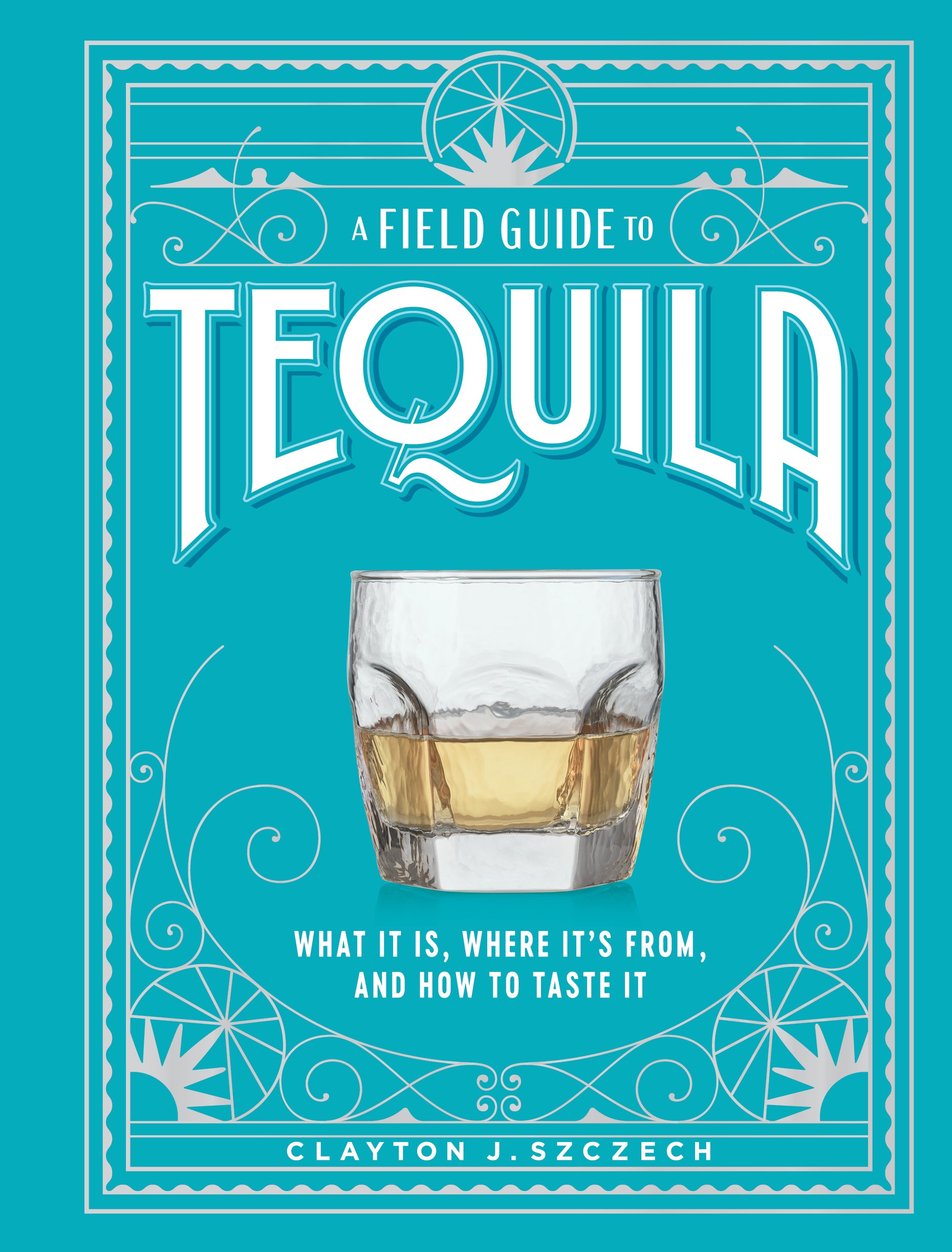This detailed book cover showcases "A Field Guide to Tequila," centrally positioned and prominently displayed in large white letters. Below the title, the subtitle elaborates on "what it is, where it's from, and how to taste it." The cover is a striking medium teal blue, adorned with intricate white filigree and abstract borders that give it a vintage appeal. At the center of the cover, there is a small clear glass, about two inches tall, filled halfway with light beige, aged tequila. The author's name, Clayton J. Szyszek, is neatly situated towards the bottom of the cover in matching white font, adding to the overall elegant and informative design.